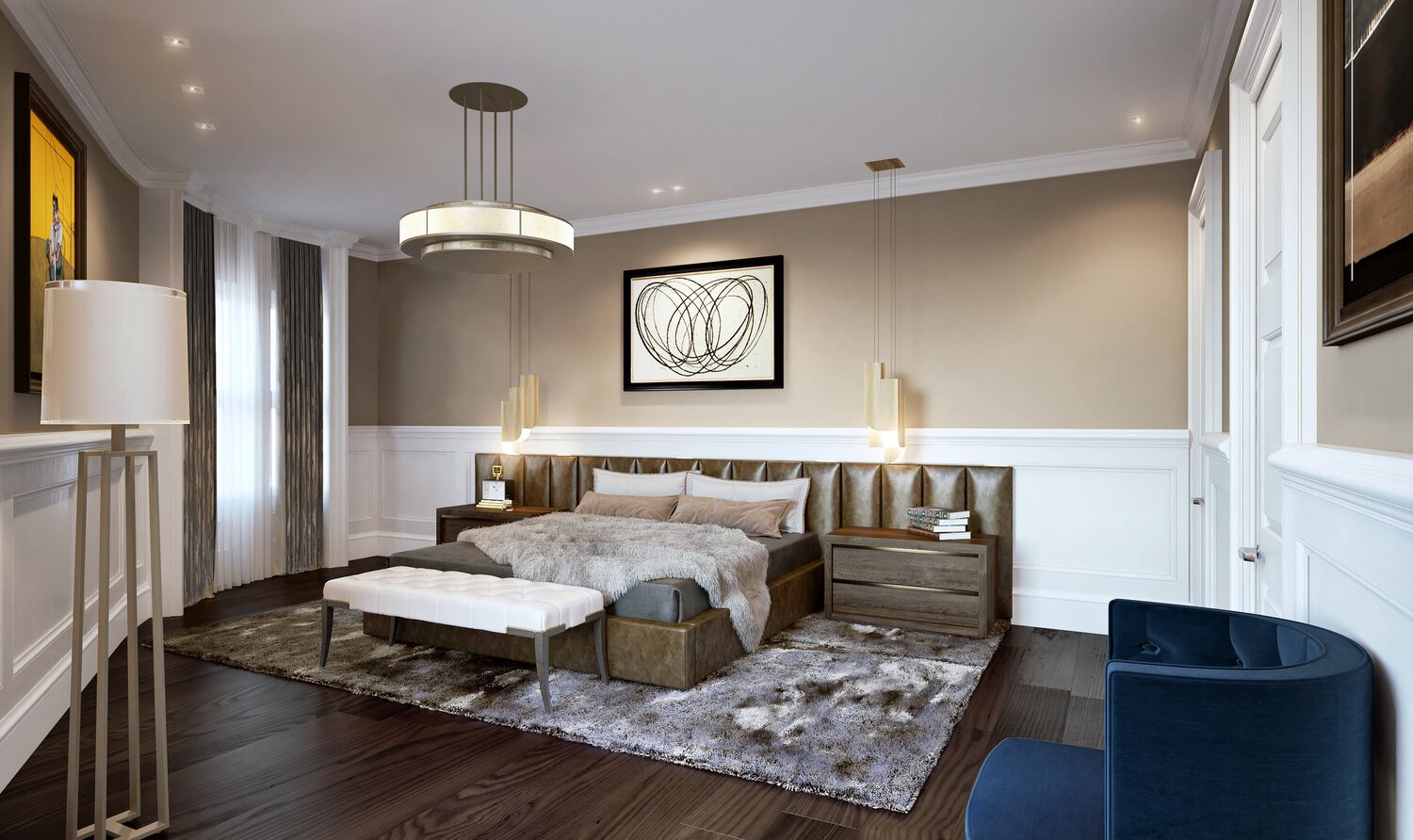This detailed 3D color illustration rendering depicts the modern-natural interior of a beautifully designed bedroom. The centerpiece is a bed with a patent leather headboard featuring vertical stitching, flanked by dark brown wooden nightstands. Above the headboard, a minimalist artwork with a black frame and a swirling circular design on a cream background draws attention. The bed itself is dressed in gray sheets, a fur afghan throw, and a mix of white and beige pillows. At the foot of the bed, a white cushioned ottoman sits on a gray splotched fur area rug.

On either side of the bed, gold square pendant lamps with a mission or 1960s prairie style hang from power cables, complemented by recessed lighting in the ceiling. Additional lighting includes a white drum-shade floor lamp in the bottom left corner, standing in front of a small artificial mantel. Along the left wall, tall ceiling-to-floor draperies in dark olive frame the windows, enhancing the room's overall elegance.

The walls feature white paneling on the lower half and a soft taupe paint on the upper half. The room also includes a navy circular side chair on the right side and a creative, colorful chair rail. The dark brown wood laminate flooring adds warmth to the space, tying together the modern aesthetics with natural tones. Books and a few other personal touches on the nightstands add to the welcoming, lived-in feel of this well-appointed bedroom.